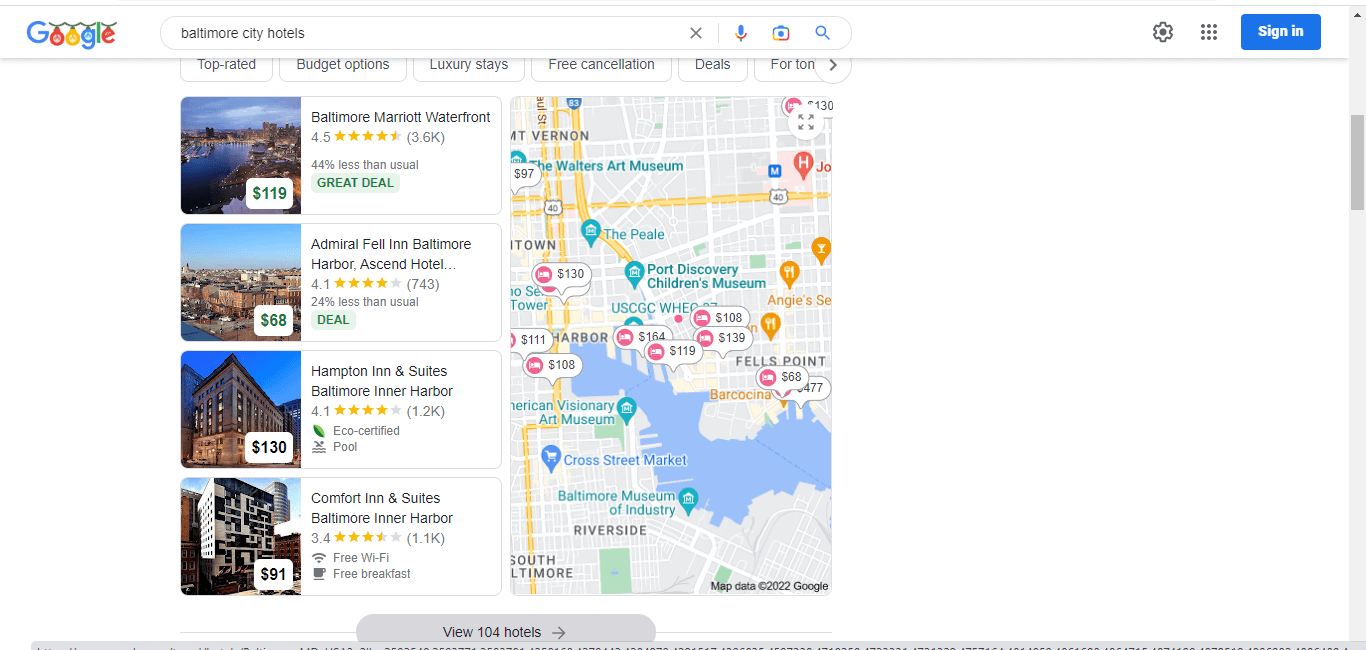A screenshot of a Google search for "Baltimore City Hotels" on a computer screen. The Google logo at the top of the page features a blue capital 'G', followed by an 'o' in red, another 'o' in yellow, a 'g' in blue, an 'l' in green, and an 'e' in red. The letters appear arranged in a way that makes them look like they are hanging from strings, reminiscent of Christmas ornaments. Below the search bar, the image displays four hotel search results on the left-hand side, partially cut off at the bottom. 

1. **Baltimore Marriott Waterfront**:
   - Rating: 4.5 stars
   - Price: $119 per night
   - Note: "Great deal"

2. **Admiral Fell Inn Baltimore**:
   - Rating: 4.1 stars
   - Price: $68 per night
   - Note: "Deal"

3. **Hampton Inn & Suites Baltimore Inner Harbor**:
   - Rating: 4.1 stars
   - Price: $130 per night
   - Note: "Eco Certified Pool"

4. **Comfort Inn & Suites**:
   - Rating: 3.4 stars
   - Price: $91 per night
   - Amenities: Free Wi-Fi and Free Breakfast

On the right-hand side of the page, a map displays the locations of these hotels within Baltimore.